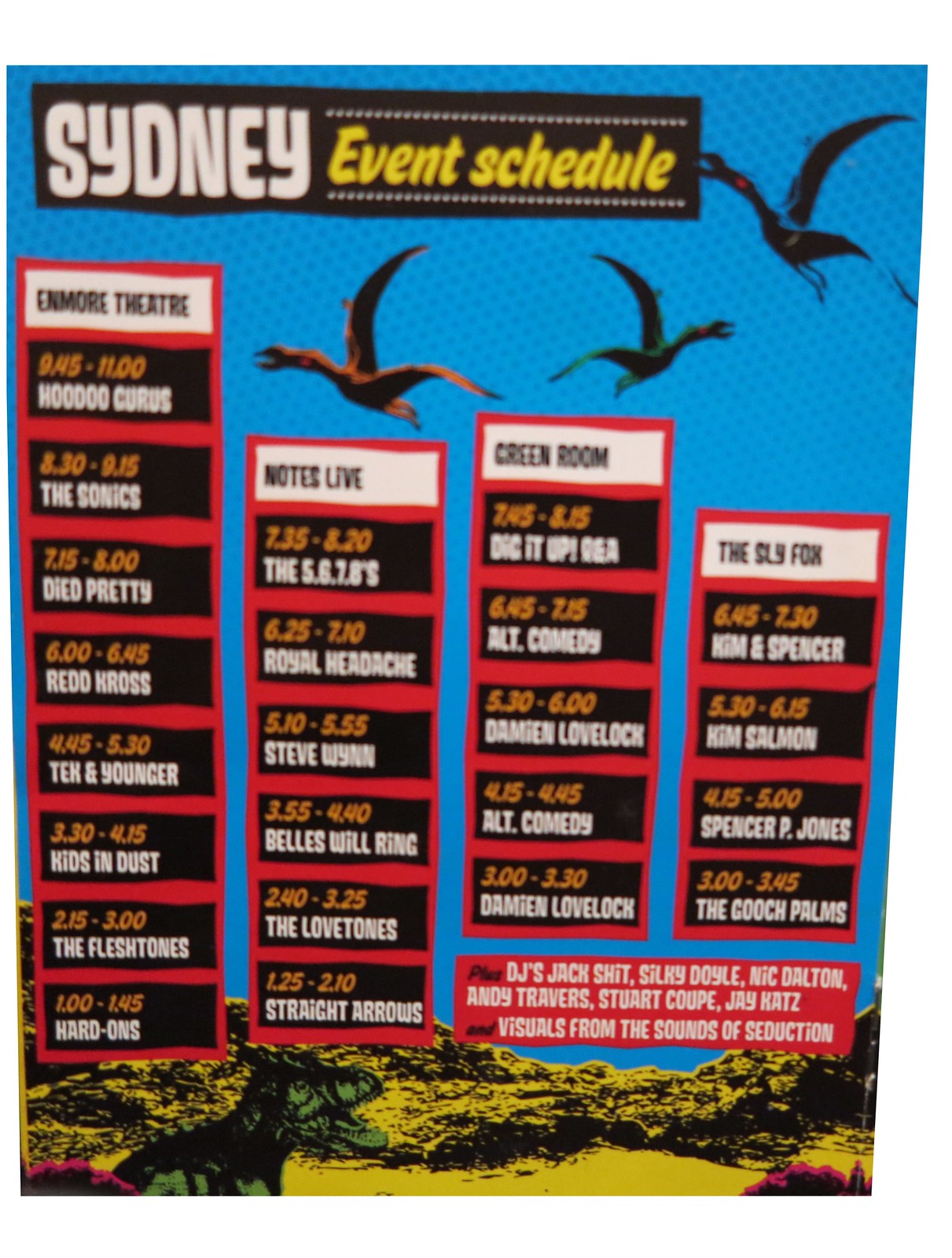The poster titled "Sydney Event Schedule" features a vibrant and detailed layout. At the very top, against a sleek black bar, the words "Sydney" appear in bubbly white text, while "Event Schedule" is written in slanted yellow text. Below this, set against a bright sky-blue background, float three pterodactyl-like dinosaurs, suggesting a prehistoric theme. A Tyrannosaurus Rex or similar dinosaur is subtly visible at the bottom of the poster, adding a hint of ferocity to the image.

The schedule itself is divided into four horizontal columns, each headed by a different venue name and listed with events. The columns are outlined in vivid colors to distinguish each venue. The first column, titled "Amor Theatre," lists performances by artists such as Who's Circus, The Sonics, Died Pretty, Red Cross, Tech and Younger, Kids and Dust, and The Fleshtones. The second column, "Notes Live," catalogs events at specified times. The third, "Green Room," and the fourth, "The Sly Fox," similarly enumerate events hosted at those venues.

The events are listed in black boxes, with event times highlighted in orange. Detailed descriptions of each event are provided in white text beneath the time listings. The ground of the poster features a lime-green grassy hill casting a black shadow, completing the engaging and dynamic design.